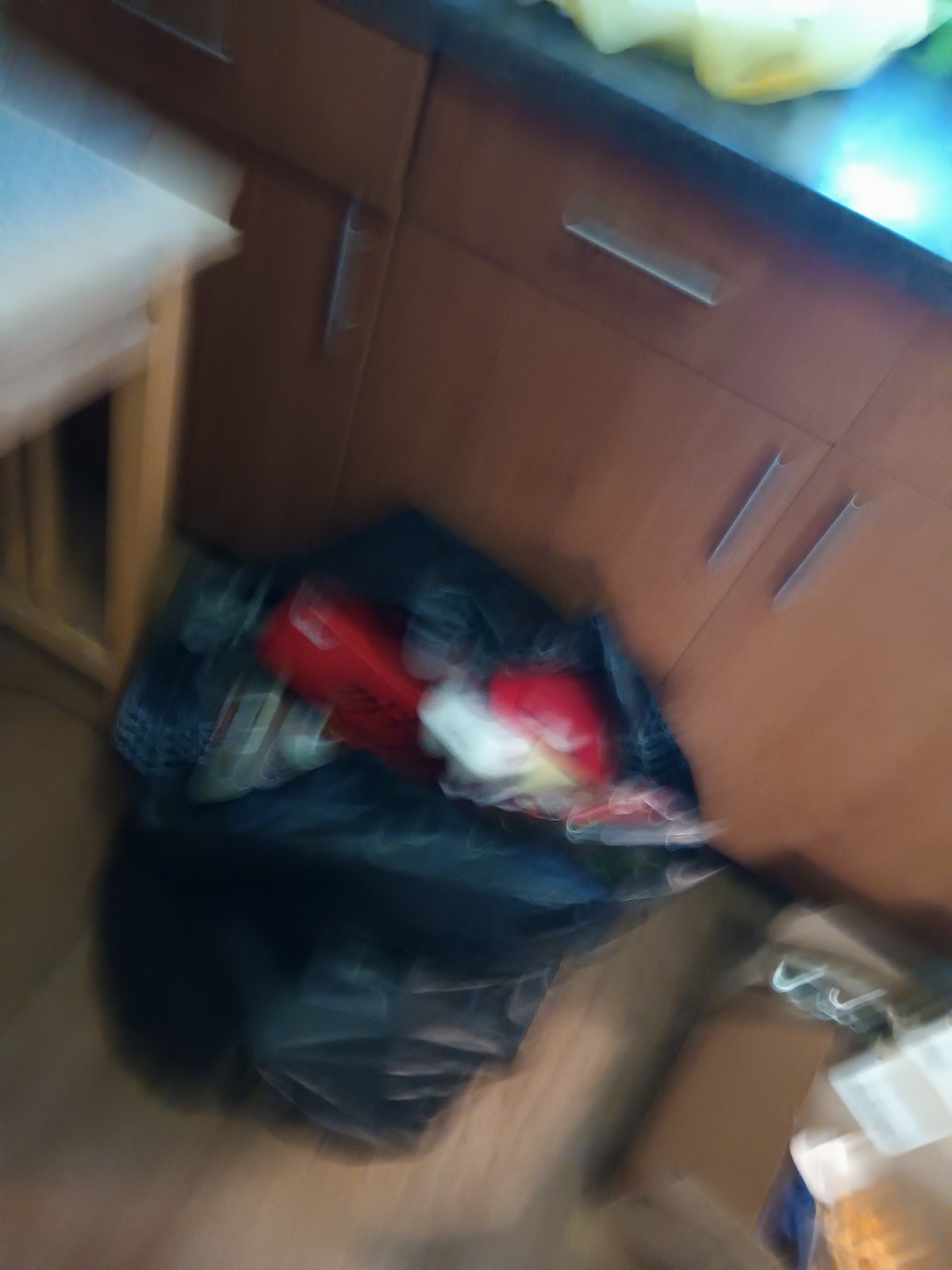The image in question is a portrait-oriented, somewhat blurry photograph capturing a scene likely set in a kitchen. The focus of the image is a person, partially visible, leaning over and looking down at either a garbage can or a black garbage bag filled with various discarded items. Among the visible trash, one can discern what appears to be plastic red cups and other common waste items. In the background, there's a glossy black countertop with cabinet doors underneath. In the bottom right-hand corner, there are one or two small cardboard boxes, partially visible. The upper left corner of the image shows the edge of a white tabletop supported by beechwood-colored legs. The scene suggests a moment of cleaning or tidying up in a kitchen environment.